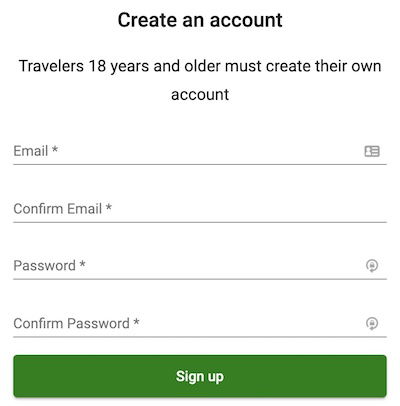The image depicts a website with a white background where a user is in the process of creating an account. At the top of the page, there is a bold heading that reads "Create an Account," with a capital "C." Just below the heading, text in a darker shade informs, "Travelers 18 years and older must create their own account," with the number 18 in numeric form and a capital "T" for "Travelers."

The form consists of four horizontal fields, each with a gray background. The first field is labeled "Email*" in gray placeholder text, with "Email" starting with a capital "E" and an asterisk denoting a required field. To the right of this field, there is an ID icon displayed as a gray silhouette of a head and shoulders, accompanied by three white horizontal lines suggesting a user profile.

The second field below is labeled "Confirm Email*" with both "Confirm" and "Email" capitalized, again indicating a required field with an asterisk.

The third field is labeled "Password*" with a capital "P" for "Password." On the far right side of this field, there is a lock icon featuring a line and arrow encircling it, symbolizing security.

The fourth field, "Confirm Password*," follows the same format, with capitalized words and an asterisk, and includes the same lock icon on the right.

Beneath these fields, there is a conspicuous green button with the text "Sign Up" in white and a capital "S" for "Sign," inviting the user to complete the account creation process.